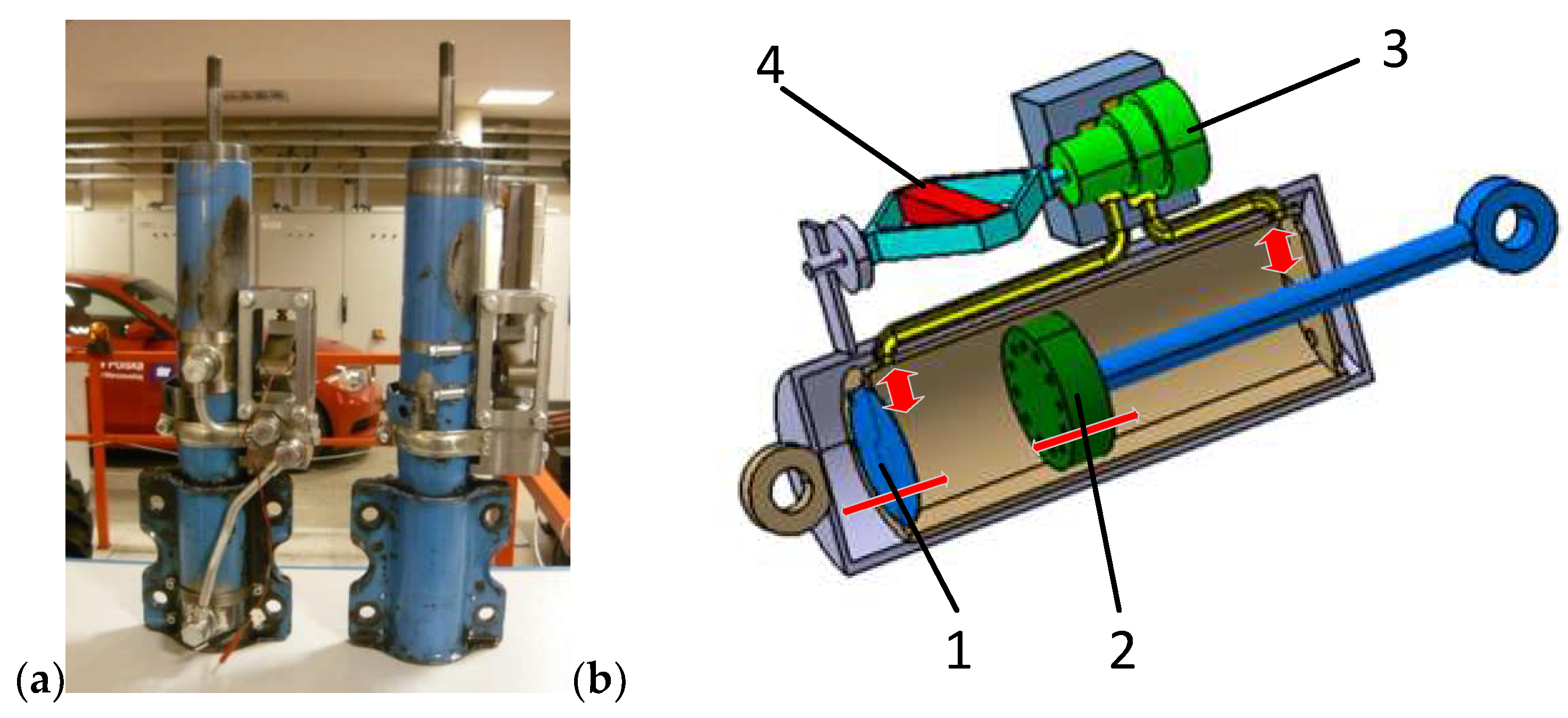This image, set against a plain white background, features two side-by-side illustrations — a photograph on the left and a detailed drawing on the right. The photograph on the left, roughly taken in an indoor factory environment, shows a sophisticated piece of machinery. In the background, there's a red automobile, suggesting an automotive context. In the foreground, mounted on a raised platform, stand two large blue canisters, likely pumping devices, each with a metal pipe extending from the top. These canisters are secured with U-bolts and feature a silver brushed metal brace connected to their sides. The canisters connect to hoses at both the upper and lower sections.

Adjacent to the photograph, the drawing on the right offers an internal view of one canister, showcasing its intricate components which include a hydraulic press and a cylindrical plunger mechanism, labeled numerically for clarity. The plunger moves within the canister, appearing to control air or fluid flow, while different segments depict interconnected hoses and a bulkhead that moves back and forth. Unlike the photograph, the drawing provides clear cross-sectional insight into the internal workings of the machinery, including labeled elements like a green cylinder at the bottom and a diamond-shaped flex steel component related to the pulley system.

Overall, this juxtaposed display of the machinery in real and illustrated form highlights the technical complexity of the pumping devices, with the photograph capturing the external assembly and the drawing elucidating the internal mechanisms.